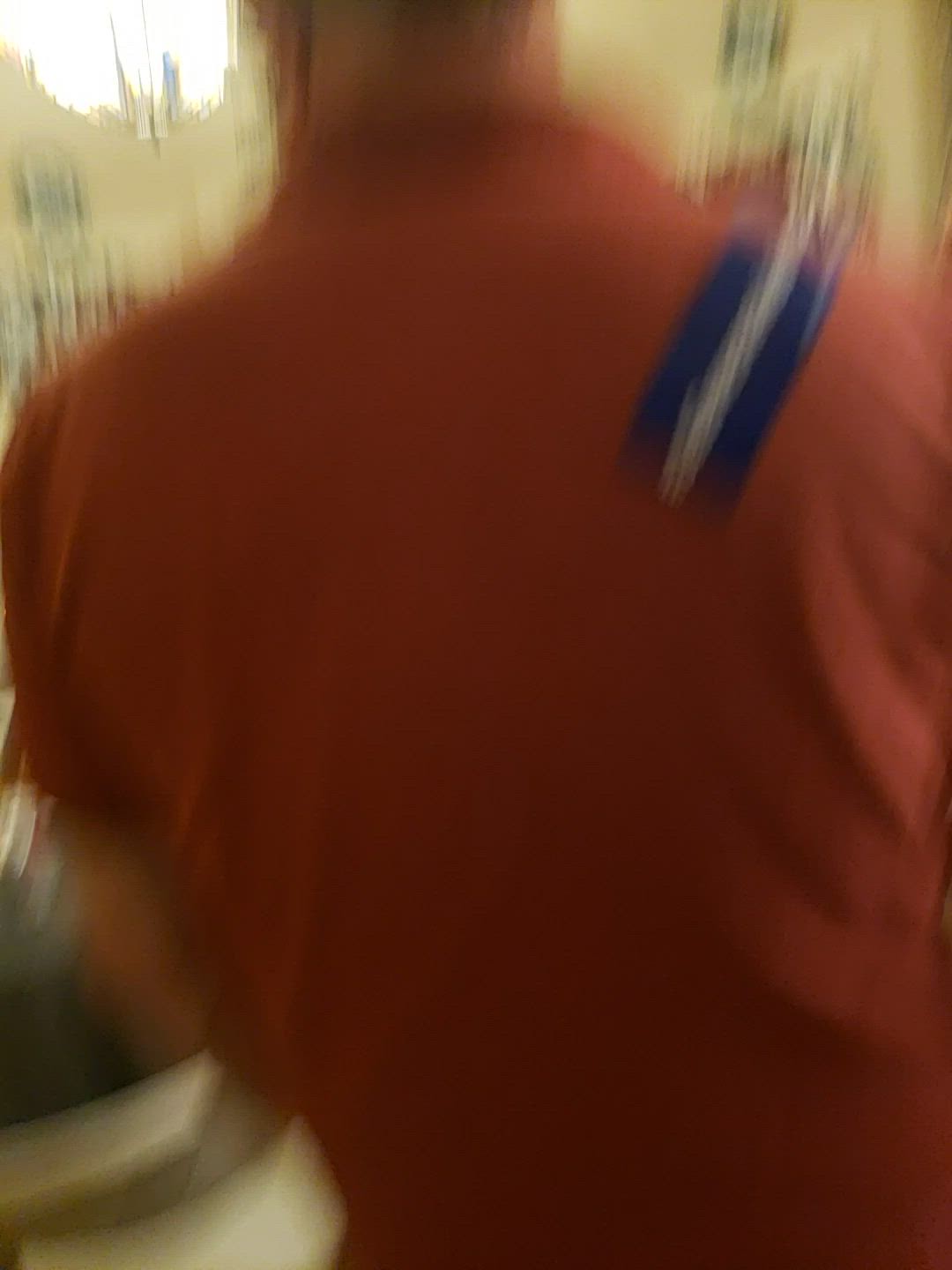A large man stands prominently in the center of what appears to be a spacious living room. He is dressed in a bright pink shirt which features a blue patch on the back with indistinct, blurred text. The room is well-lit, potentially from a window at the top of the image, allowing natural light to flood the space. At the bottom of the image, a plant is visible, adding a touch of greenery to the setting. The white walls are adorned with pieces of art or decorative items. The overall ambiance suggests a cozy and personalized living area within a home.